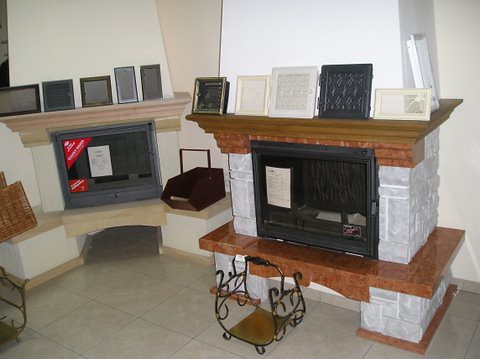In a showroom setting, a digital photograph captures two fireplaces against a slightly cream-colored back wall, highlighting the contrast between their designs and finishes. Both fireplaces feature wooden mantels, with the farther fireplace adorned in a natural tan color, while the nearer one has dark brown mantels. The left, corner-style fireplace showcases a tan mantel with a gray insert and a red triangle sticker in its upper corner. It sits in an off-white chimney structure with a decorative wicker basket nearby. The right fireplace, crafted from white-painted faux brick, features a black insert encased in an unattractive rusty stone surround and a matching wrought iron log holder in front, its mantelpiece topped with empty picture frames. The floor, tiled in a cream shade, unifies the space, emphasizing the functional yet diverse stylistic approach to fireplace design.